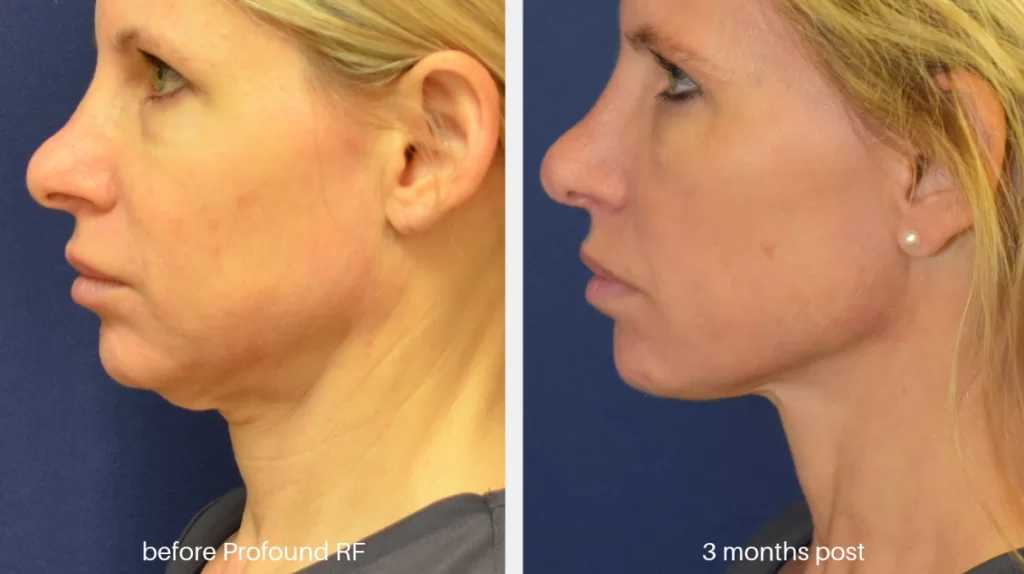The image is a side-by-side collage of a middle-aged woman's before and after results of a treatment, likely Profound RF. On the left, the "before" photo shows the woman with blonde hair, a fair complexion, and she dons a dark shirt visible only at the base of her neck. She has a round face with a double chin and wrinkles, offering a stern expression. The "before profound RF" text is located at the bottom. On the right, the "after" photo, taken from the same angle and seemingly with the same shirt, depicts the woman three months post-treatment. She now exhibits a slimmer face with a sharper jawline, reduced wrinkles, and a more defined facial structure. Notably, she also wears an earring in this photo. The overall transformation highlights significant improvements in her chin and neck areas.